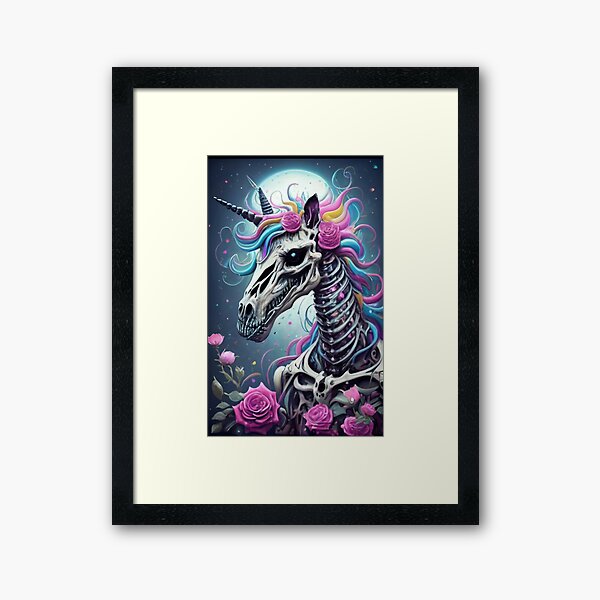The image features a color photograph of a framed and matted piece of artwork. The frame is black with a cream-colored mat, housing a drawing that intricately combines elements of fantasy and horror. At the center of the artwork is a bipedal skeleton of a unicorn, depicted from the torso upwards, standing upright against a backdrop of a full moon and a starry sky. The skeleton bears the head of a horse but with a prominent unicorn horn, and it features menacing teeth and a dark, black eye peering from its skull. Flowing pastel-colored hair—including hues of light blue, pink, yellow, and teal—adorns the unicorn's head, drifting between its ears and the back of its neck. The scene is made even more surreal and engaging with the presence of purple and pink roses scattered around the unicorn and incorporated into its mane, lending an eerie yet whimsical touch reminiscent of H.R. Giger’s style.